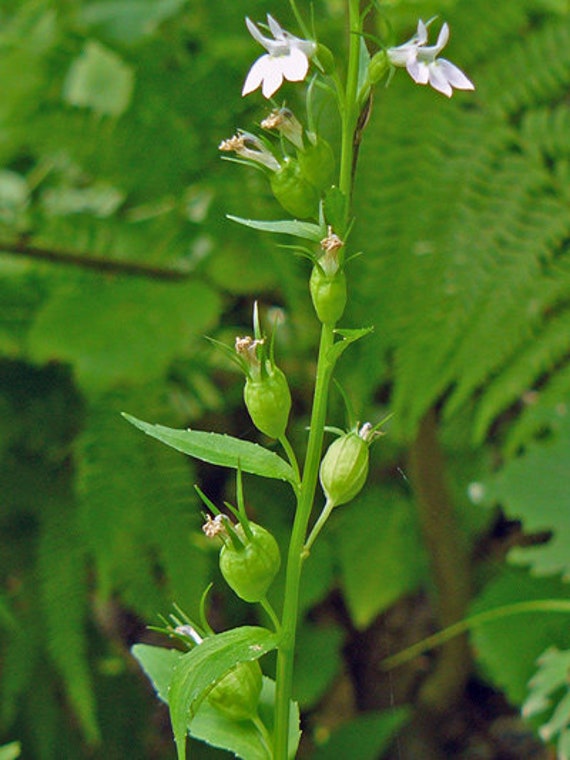In this outdoor image, the background is softly blurred, revealing an abundance of green foliage and ferns, likely from various shrubs. These verdant leaves create a lush, textured backdrop. In the foreground, a singular plant stands in sharp focus. The plant has a green stalk adorned with slender, pointed leaves. Emerging from the stalk are small, bulb-like structures, which appear to be the pods of flowers yet to bloom. These pods are green, with tinier, needle-like leaves sprouting from them. At the top of the plant, several white flowers have fully blossomed, their petals spread out evenly and delicately, adding a touch of purity to the scene. A close inspection reveals a particular flower with a hint of whitish-purple, contrasting the otherwise predominant green hues.